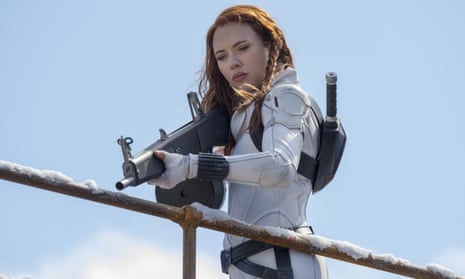In an outdoor setting under a light blue sky with scattered clouds, a young woman in her 20s stands poised. Her striking appearance features long red hair, partly braided on one side and loose on the other. She dons a sleek, white jumpsuit complemented by white gloves with black bands around the wrists, and a black belt cinched at her waist. A black backpack with a protruding, stick-like projection rests over her left shoulder. The woman possesses a serious expression, her eyes almost closed but intensely focused as she aims a large, black machine gun downward. To her side, a handrail dusted with snow runs horizontally across the scene, intersected by a single vertical pole. The overall composition evokes a sense of a futuristic or action-packed narrative, possibly from a movie.